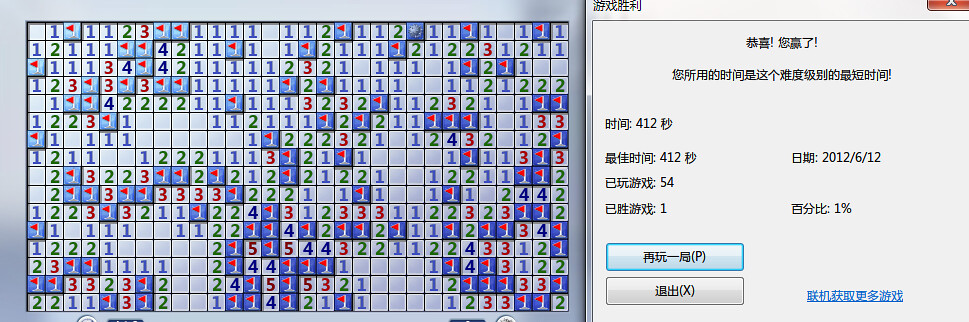The image is a detailed screenshot of a Minesweeper game in progress on a computer screen. The left side of the screenshot showcases the Minesweeper grid, filled with numerous squares. The grid features numbers, primarily ranging from 1 to 5, and several squares displaying red flags against a blue background. Some of the squares remain blank, indicating unexplored areas. On the right side of the image, there is a pop-up window with text in Chinese characters, making it unreadable for those unfamiliar with the language. This pop-up window also includes two buttons, one blue in the top left and the other gray, along with an underlined, blue hyperlink. Notably, the date "2012/6/12" is visible within the window.